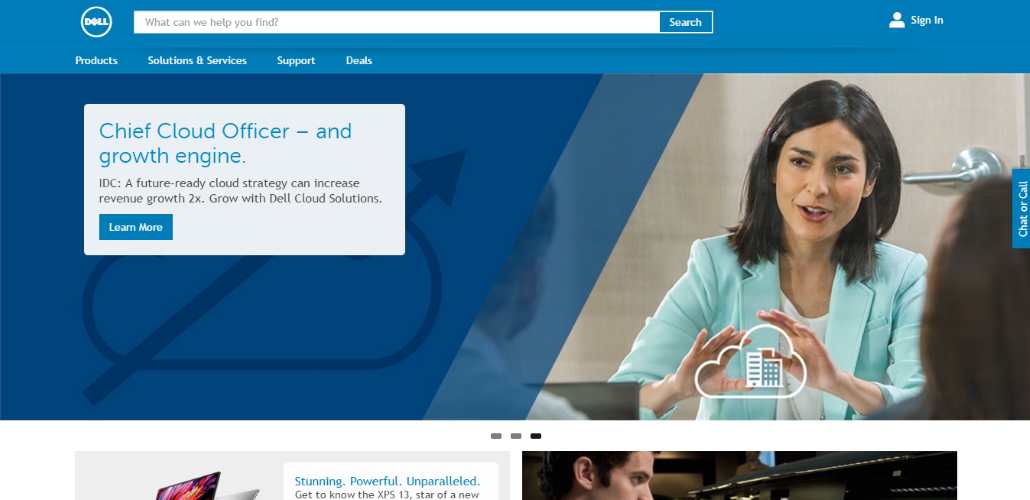The webpage is from the Dell official website, prominently featuring the word "DELL" in white, capitalized letters enclosed within a white circle, situated atop a blue navigation bar. Just beneath this label, there's an extensive white search bar with placeholder text in gray font reading, "What can we help you find?" Adjacent to this, on the right-hand side, lies a distinctly blue search button with white text. There's also a white icon for user sign-in on the far right of the header.

Below this, there's another blue bar, matching the color of the top navigation bar, displaying white text for different sections: "Products," "Solutions and Services," "Support," and "Deals."

The main body of the webpage features a large image on the left side. This background image is predominantly blue, depicting a circular arrow pointing upwards to the right, though partially obscured by a white box. Inside this white box, there is blue text that reads, “Chief Cloud Officer - Growth Engine.” Beneath it, in black font, is a text stating, “IDC: A future-ready cloud strategy can increase revenue growth two times. Grow with Dell Cloud Solutions,” followed by a clickable blue button with white text that says, “Learn More.”

To the right of this image, there is a photograph of an attractive woman with shoulder-length, straight black hair, wearing a seafoam green jacket over a white shirt. She appears to be speaking with her mouth slightly open and has her hands raised in front of her. Visible in the background are parts of two other individuals - on the right, the back of a man's head, and on the left, another woman with long dark hair. Between the woman’s hands, there is a small white cloud icon.

Below this main section, the tops of two additional images are visible. The left image shows part of a Dell computer with blue text declaring, “Stunning, Powerful, Unparalleled” followed by gray text, “Get to know the XPS 13.” The right image is darker, showing a side profile of a man’s head, revealing his ear, eye, and nose. The man appears to have short dark hair and light skin.